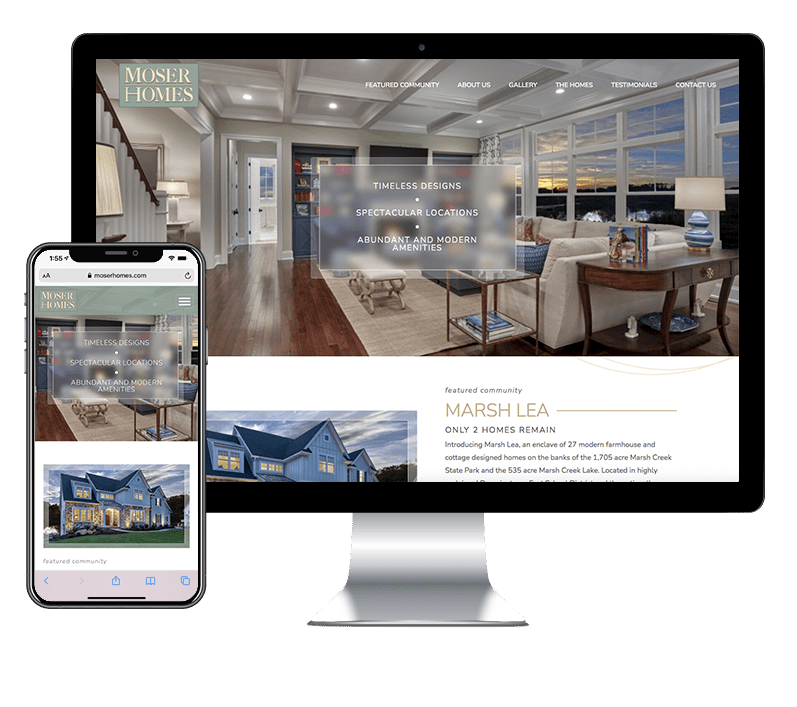The image showcases a detailed screenshot of the Moser Homes website as displayed on both a desktop computer and a mobile phone. Although it is not a literal photo of the devices, the screenshot effectively illustrates the website’s responsive design and user interface. 

On the desktop view, the website features a prominent header with a navigation menu that includes sections such as "Featured Community," "About Us," "Gallery," "The Homes," "Testimonials," and "Contact Us." This menu highlights the extensive information Moser Homes provides about their properties and services. 

The main content area beneath the navigation menu prominently displays the taglines "Timeless Designs," "Spectacular Locations," and "Abundant Modern Amenities." These phrases underscore Moser Homes' emphasis on luxury, modern design, and premium locations. The overall presentation suggests an aim to appeal to discerning clients seeking high-end residential options with contemporary conveniences.